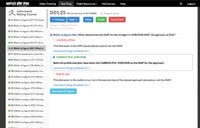The image depicts a distant and somewhat indistinct view of a webpage. The page is divided by a prominent black vertical line on the left side, extending from the top to the bottom. On the right, there is another vertical line that is slightly shorter at the bottom and thinner than the one on the left. At the top of the page, a horizontal black line stretches across from left to right, appearing to be of similar, if not slightly greater, width compared to the left vertical bar. This horizontal line contains some white text that is illegible due to the distance. Below this, the page is structured into sections, with the leftmost section followed by six more segments containing unreadable white words. Beneath these sections, there is a numerical figure, followed by a sequence of three blue Bluetooth icons or buttons.